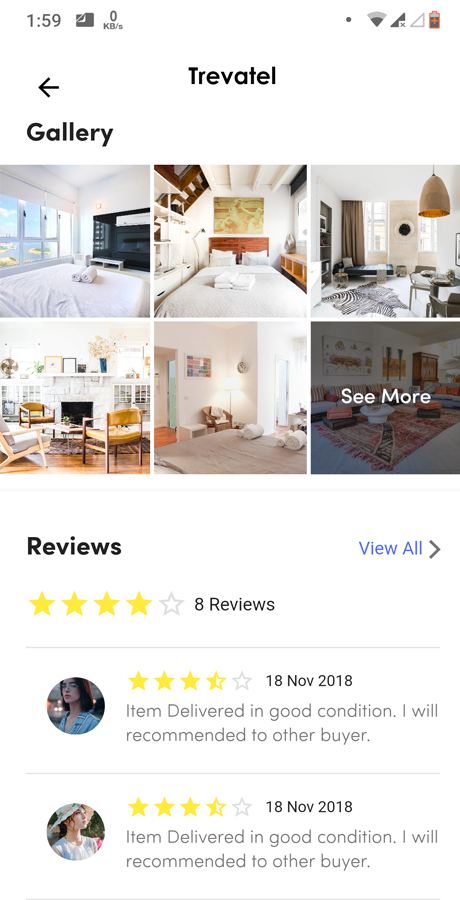This image depicts a screen capture from the website Truebottle. At the very top, the status bar shows the time as 1:59, alongside icons for cellular signal, Wi-Fi, and battery status positioned on the upper right. Below this, the Truebottle logo is centrally placed in bold black text. On the upper left, a back arrow is visible, with the word "Gallery" written beneath it.

The main section of the screen showcases a gallery of six images arranged in two rows of three. These images appear to be of hotel rooms or homes. Notably, the last image on the bottom right has an icon or cover indicating it can be pressed for more information.

Further down, the "Reviews" section is displayed, with a "View All" button on the right-hand side. This section reveals that there are a total of eight reviews, with an average rating of four out of five stars. The first two ratings visible are both three and a half stars. The associated review text reads: "Item delivered in good condition. I will recommend to other buyers," and this same review is repeated for the second rating.